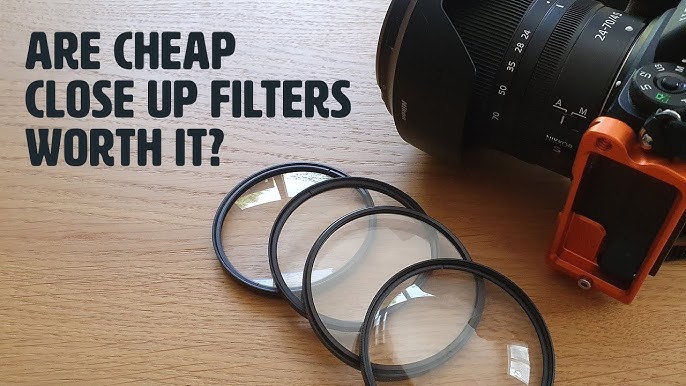In the image, a light brown, artificial wood table serves as the backdrop for a carefully arranged display of a traditional film camera and four close-up filters. The camera, which is predominantly black with a bright orange attachment on one side, features various detailed markings, including numbers like 70, 50, 35, 20, and 8, as well as 'A' and 'M' settings indicative of automatic and manual modes. The four filters, with their clear lenses and black rims, are positioned to the left of the camera. One filter lies flat on the table, while the remaining three are propped up sequentially, creating a domino-like effect. Reflections in the filters suggest a windowed setting. In the upper left corner of the image, bold black text in a Comic Sans-like font poses the question, "Are Cheap Close-Up Filters Worth It?" The overall composition and style suggest this could be an advertisement, a social media post, or a thumbnail image.